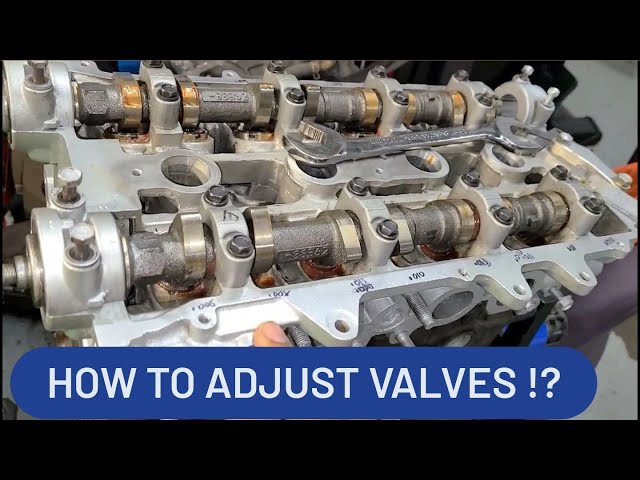This image captures a detailed, close-up view of an exposed engine's internal components, specifically showcasing two rows of four metal cylindrical objects within a larger light gray metal framework from an overhead perspective. Notably, a double-sided wrench rests on top of the machinery, suggesting ongoing maintenance work. The image is framed in a horizontal, rectangular format with black borders at the top and bottom, reminiscent of a widescreen video still. At the bottom of the frame, a blue, ovular border features white uppercase text that reads, "HOW TO ADJUST VALVES!?" Additionally, a fingertip is visible, reaching up from the bottom edge just above the text, hinting at human interaction with the machinery. The dominant colors in the image are metallic silvers, older bronze tones, and black. There are also partial glimpses of other individuals around the edge of the motor, indicating that the scene involves multiple people. The combination of these elements suggests that this is likely a thumbnail or screen capture from an instructional video on engine maintenance.